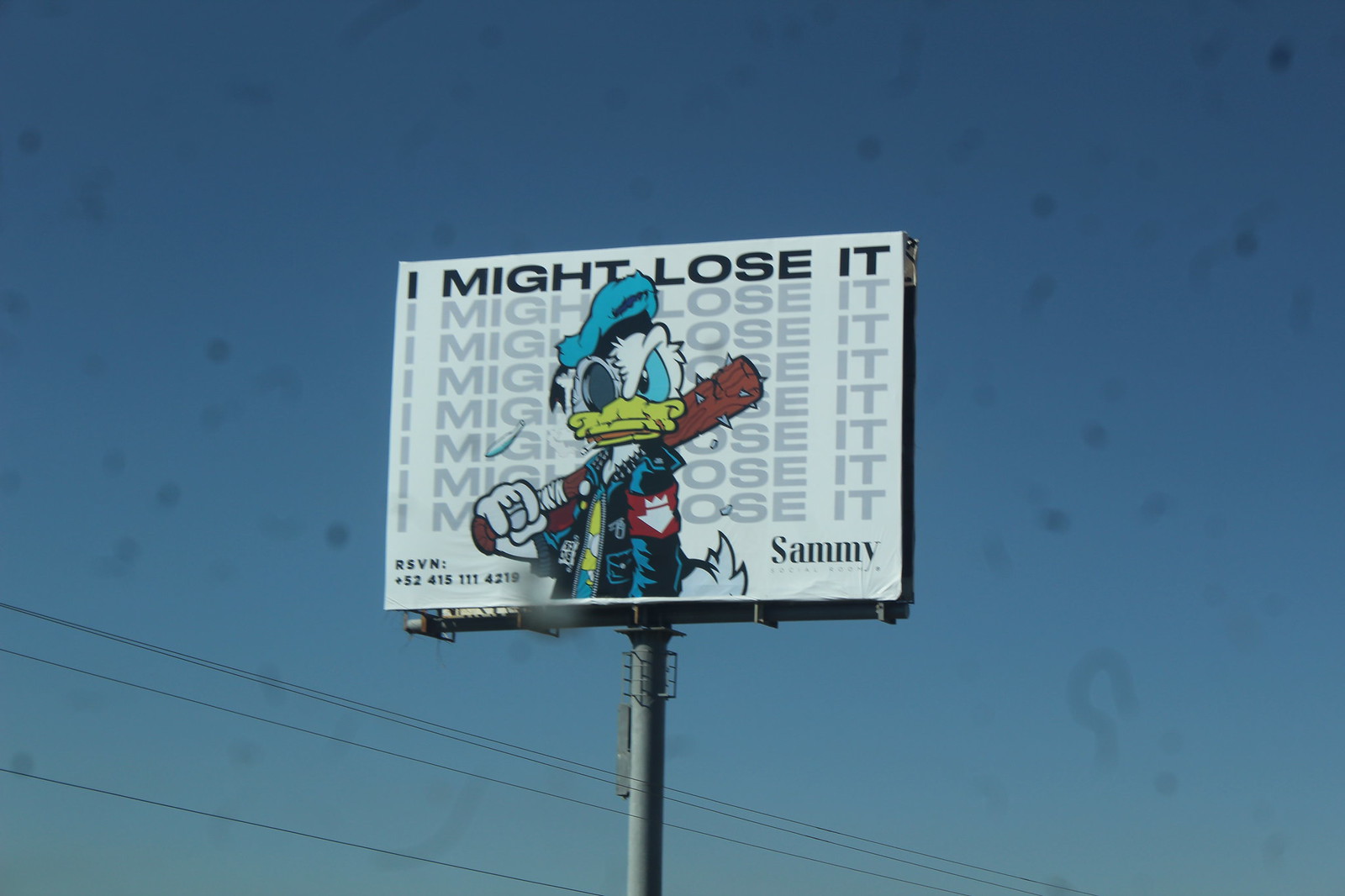This image depicts a tall roadside billboard perched on a wide, metallic pole, towering above visible power lines. The sky around the billboard is a vivid blue. The billboard itself is predominantly white and features a menacing depiction of Donald Duck, who appears disheveled and hostile. He sports an eyepatch, a leather jacket, and holds a spiked bat, evoking a tough, gang-like appearance. Boldly written in black at the top, and then repeatedly fading to gray, are the words "I might lose it," echoed seven more times behind Donald. The name "Sammy" is positioned in the bottom right corner, accompanied by a phone number with a country code of 52. The photograph was taken from behind a dirty vehicle windshield, which is evident by the visible spots on the glass.